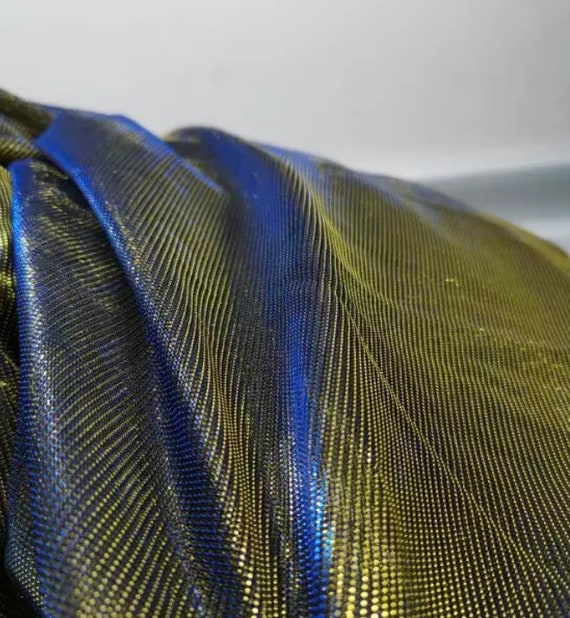This image features a close-up view of a colorful, metallic-like fabric that occupies roughly three-quarters of the picture, with a plain white background above it. The fabric has a textured, leathery appearance and is folded haphazardly, creating three distinct creases that run from left to right. The material reflects light in various hues, primarily showcasing a mix of blue, gray, yellow, black, and hints of teal and lime green, lending it a shimmery, ethereal quality. The surface of the fabric is adorned with numerous small, dot-like textures that resemble tiny gold points or scale-like patterns, adding to its intricate appearance. These dots contribute to its metallic feel, reflecting the light to create a dynamic range of colors, especially at the edges where the fabric transitions from blue to black and yellow. The overall scene suggests the fabric is laid over a slightly domed object, enhancing the visibility of folds and wrinkles throughout the material.